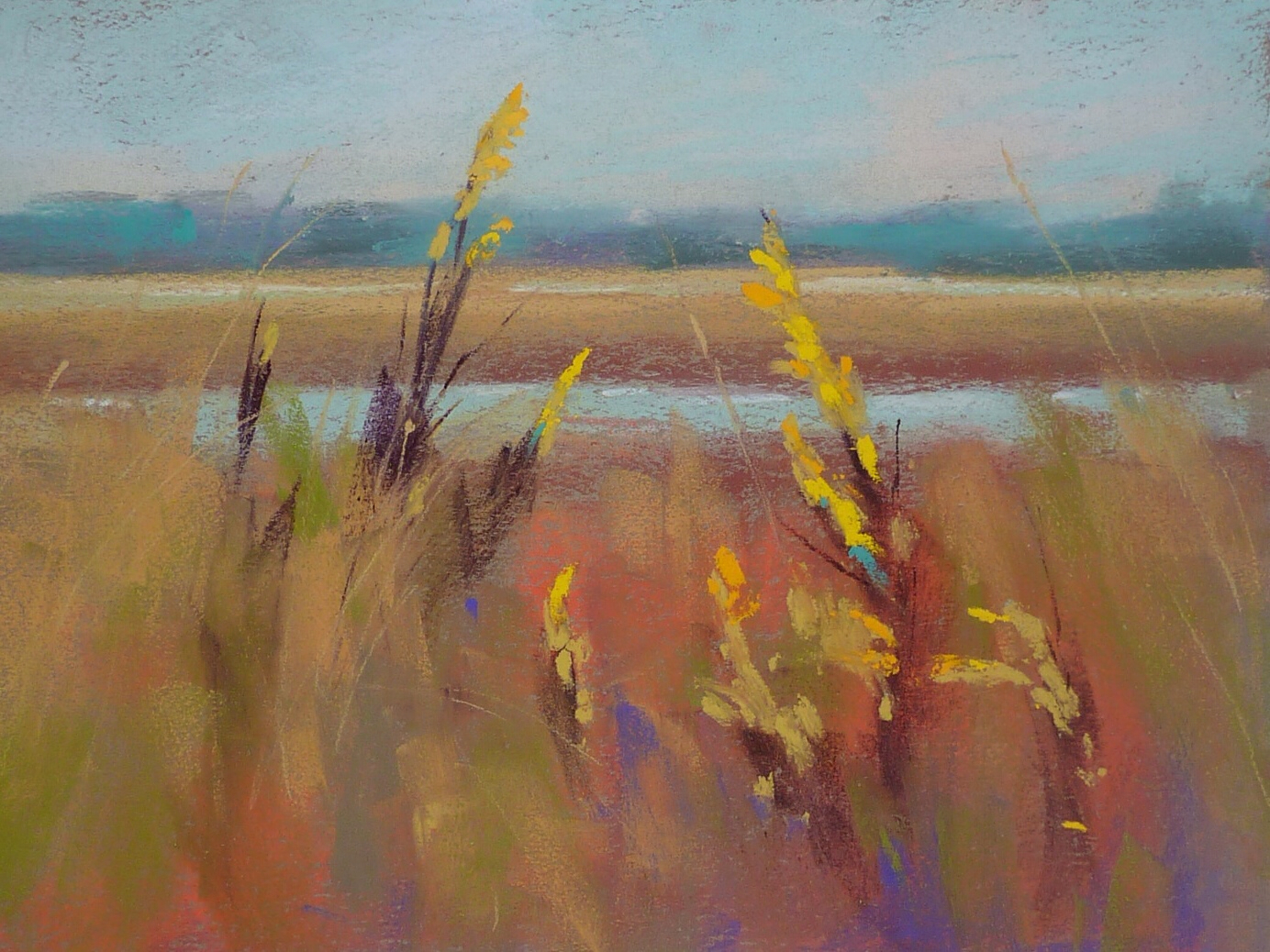This painting depicts a serene natural landscape at sunset, rendered in a dreamy, pastel-like style. The sky is a light blue with hints of pink and orange, suggesting an early sunset. Below, darkish brown, blue, and purple formations evoke distant mountains. A body of water, possibly a lake or river, runs horizontally through the middle, bordered by greenish-brown land that transitions into a lush, marshy foreground. Here, tall, yellow-stemmed plants hint at a marsh environment. The painting's impressionistic quality, perhaps achieved through watercolor or oil techniques, imbues it with a soft, blurred clarity that invites contemplation. The use of varied colors, including oranges, browns, greens, and blues, enhances the dreamlike, almost ethereal atmosphere of this natural scene.